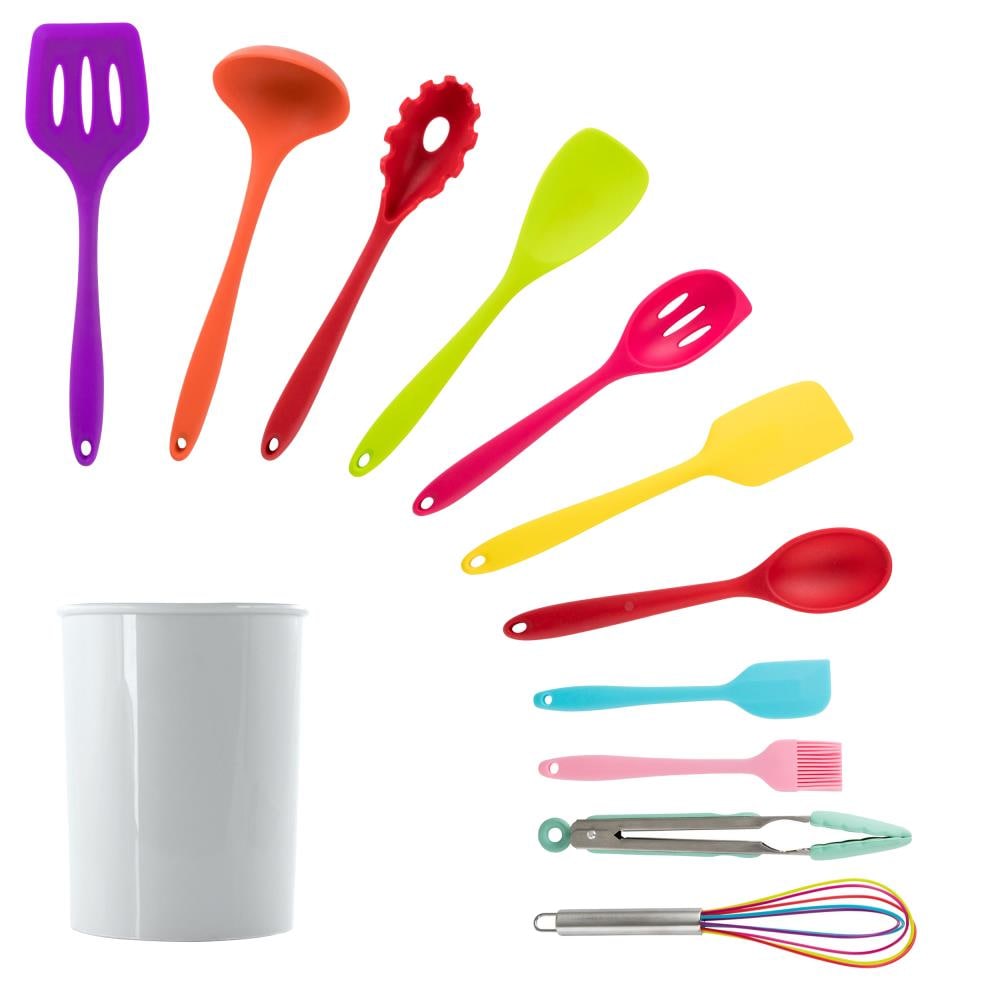The image showcases a white, shiny, cylindrical canister positioned in the bottom left corner, serving as a tool holder for an array of colorful silicone kitchen utensils. These utensils are arranged in an arch, fanning out from the top left to the bottom right against a pristine white background. Starting from the top left, the lineup includes a purple pancake flipper-style spatula, followed by an orange ladle, a red slotted spoon, then a lime green flat scraper spatula. Next is a pink spatula with holes, followed by a yellow spatula, and a large red spoon. There’s also a smaller blue spatula, a pink silicone brush for basting, and silver tongs with light blue silicone handles and tips. Lastly, a whisk with a silver handle features colorful silicone wires in blue, red, and yellow. The entire arrangement is vivid, bright, and meticulously laid out, making the colorful utensils stand out prominently against the white background.